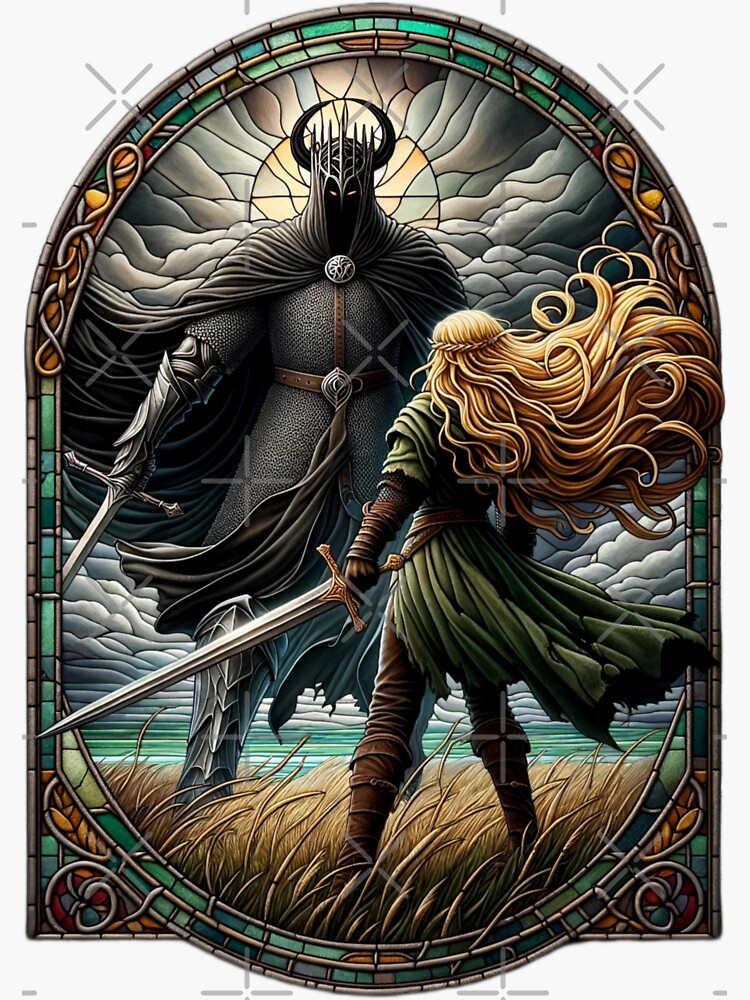This detailed color illustration, rendered in a style reminiscent of a stained glass window, depicts an epic fantasy scene. Dominating the foreground is a female warrior with long, flowing blonde hair, her back to the viewer. She is clad in an olive-colored tunic tied at the waist, brown gloves, pants, and tall dark boots. In her left hand, she wields a sword poised in a ready position. 

Facing her, in a menacing stance, is a towering, sinister figure clad in dark body armor and a black cape. This imposing adversary, partially obscured by a dark black hood, reveals only white eyes and sports devilish black horns. The figure holds a larger sword in its right hand, positioned downward.

The background unfolds as a windy, grassy plain leading to an ocean scene, with stylized clouds adding to the dramatic atmosphere. The entire scene is framed by a colorful, oval-shaped stained glass border, complete with intricate designs at the top and bottom. A radiant sun, positioned behind the black figure's head, further accentuates the stained glass effect, enhancing the image's overall fantastical and epic aesthetic.